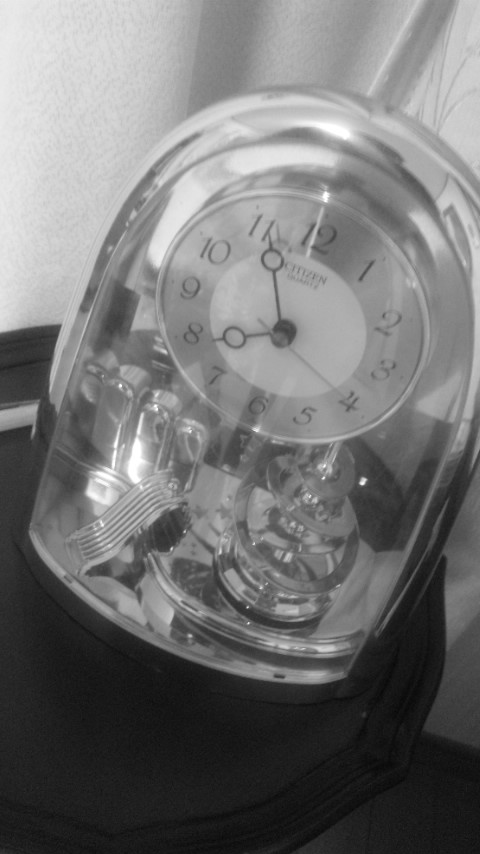This is a low-resolution black-and-white photograph of an elegant, see-through Citizen clock pointing to 7.55. The clock, designed like a dome with a flat base and rounded top, is encased in clear plastic or lucite, allowing a detailed view of the internal mechanical components. The word "Citizen" is prominently displayed behind the number 12 on the clock face, accompanied by the word "Quartz" below it. A second hand is visibly pointing to the 4. This unique timepiece, resembling a snow globe, is positioned on a small black pedestal, which could be part of a chair or a small table with a fabric-like texture. The background features a white wall and a curtain. The clock’s intricate inner workings, possibly including alarm mechanisms, are prominently visible through its transparent casing.